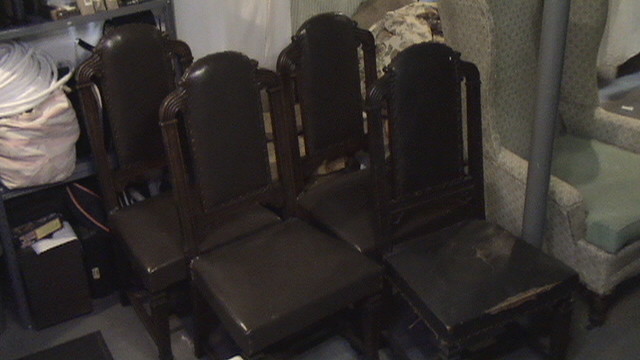The photograph depicts a storage area, possibly in a warehouse or the back of a furniture store, filled with various chairs and other items. At the center, four high-back decorative dining room-style chairs are arranged in a 2x2 configuration. These chairs are made of very dark reddish-brown, almost black, wood, with padded seats and intricately carved backs featuring scrollwork and curved tops. To the right of these, there is a high-back wing chair with a greenish-gray floral print fabric and a solid color pillow. The wing chair shows signs of wear, making it look aged and ratted. Behind these chairs, a metal storage rack with white tubing is visible, holding various items, including a black and brown top shelf, a white duffel bag on the middle shelf, and a brown suitcase and a black box with a yellow rectangle on the bottom shelf. The image also shows a vertical support post running from the floor to beyond the top of the picture frame. The floor is cement, adding to the industrial look of the setting. In the background, there are piles of white items and a small white wall. Overall, the scene suggests a cluttered storage space with a mix of antique and vintage furniture items.